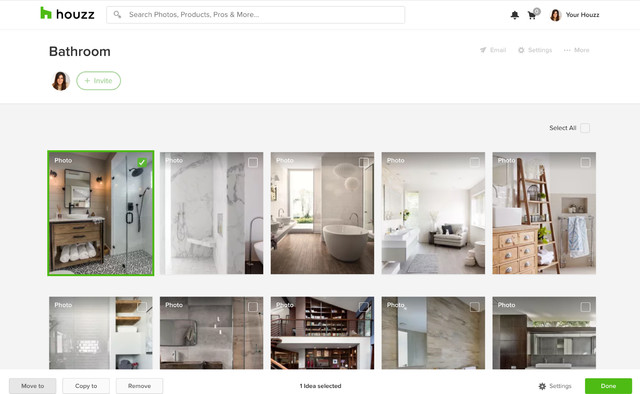The image depicts a web interface from a platform named "Houze" displayed on a computer screen. In the top right corner, there are menu options such as “Search: photos, products, pros, and more,” along with icons for notifications and a shopping cart, which is currently empty. The screen is focused on a bathroom section.

Below these menu options is a user profile section with various features like invites, email, settings, and more. The background is visually appealing, showcasing a well-designed aesthetic.

The main content displays 10 photos, with the top right image featuring a shower setup. Other images present are of wooden floors, lights, and a lighter. One of the photos includes a brick wall. Towards the bottom left of the screen, there is a gray rectangle with options such as “Copy to” and “Remove.” The interface indicates that one idea is currently selected. The bottom right side features a settings icon (gear) and a green rectangle button labeled “Done” in the middle. The entire screen is designed to help users search and manage home improvement ideas and inspirations.